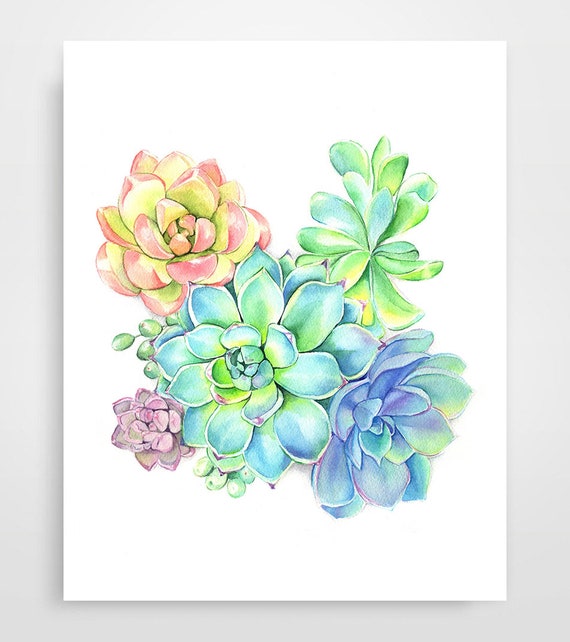The painting mounted on a gray wall is a detailed digital watercolor piece, displayed without a frame on a white canvas. This artwork features a vibrant arrangement of five distinct flowers in full bloom, each rendered in soft, blended hues of light green, blue, purple, pink, and yellow. The largest flower is centrally positioned, predominantly green with hints of blue and a touch of yellow near its center, showcasing a fully spread, vivid appearance. To its upper left, there's a sizable flower with yellow-dominated leaves transitioning to pink at the tips. Adjacent to this, in the upper right, there's a smaller, greenish stem with leaves tinged with blue. On the lower right side, a lavender and light green flower adds to the diverse floral collection. Lastly, a petite, fully bloomed pink flower with distinctly pink leaves is situated on the lower left. The leaves across all the flowers are oval-shaped with slightly pointed tips, and there are no visible seeds in their centers. The background is minimal, allowing the intricate details and delicate colors of the flowers to stand out vividly.